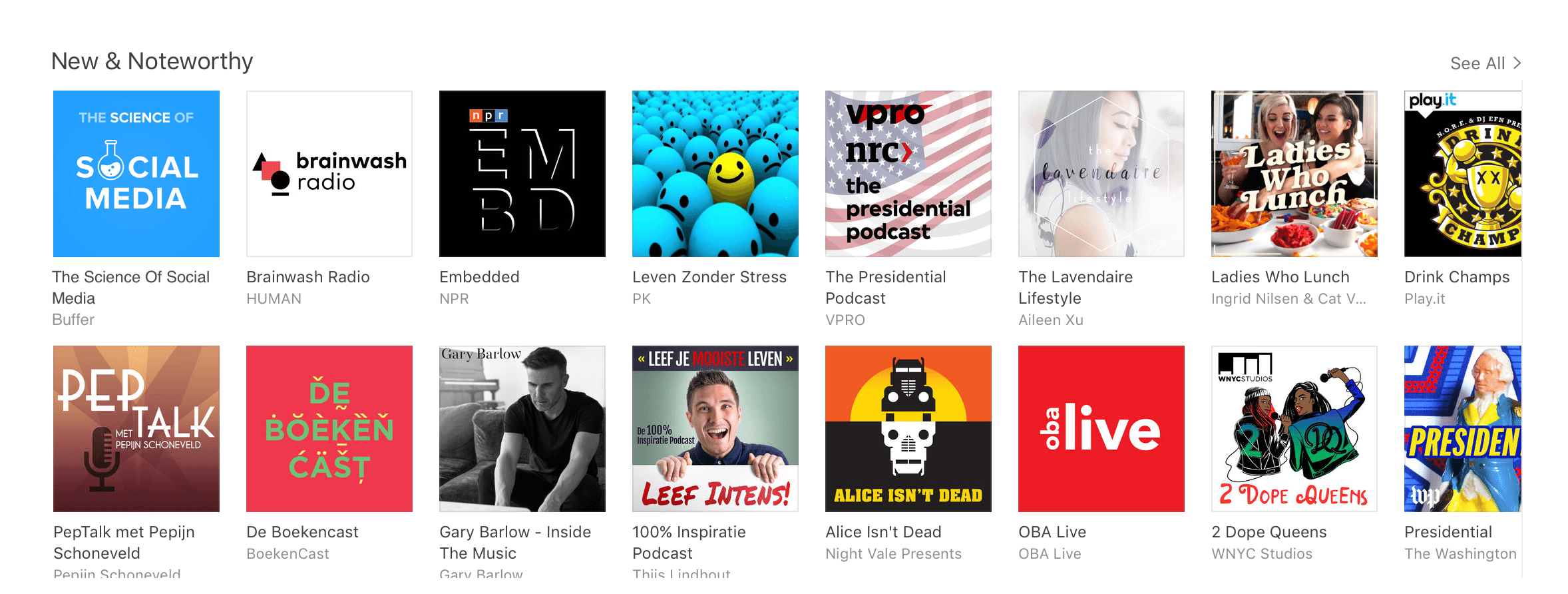This image showcases a selection of diverse podcasts under the category "New and Noteworthy." The display features two rows of podcast thumbnails, each containing eight podcasts, though the complete collection extends beyond the visible frame. Each podcast is represented by a small, colorful box with accompanying information beneath it. 

In the first row, from left to right, are the following podcasts:
1. The Science of Social Media
2. Brainwashed Radio
3. NPR Embedded
4. Leaving is Under Stress
5. The Presidential Podcast by VPRO
6. The Lavendaire Lifestyle
7. Ladies Who Lunch
8. Drink Champs

The second row includes:
1. Pep Talk
2. Dee Bokencast
3. Gary Barlow Inside the Music
4. Leaf Intends 100% in Spirit Podcast
5. Alice Isn't Dead
6. Oba Live
7. Two Dope Queens
8. Another iteration of The Presidential Podcast

Each podcast icon is uniquely designed with its own imagery and color scheme, representing a wide spectrum of colors, including black, white, gray, and almost every hue imaginable. This vibrant showcase highlights the variety and richness of the podcast realm, catering to a multitude of interests and tastes.